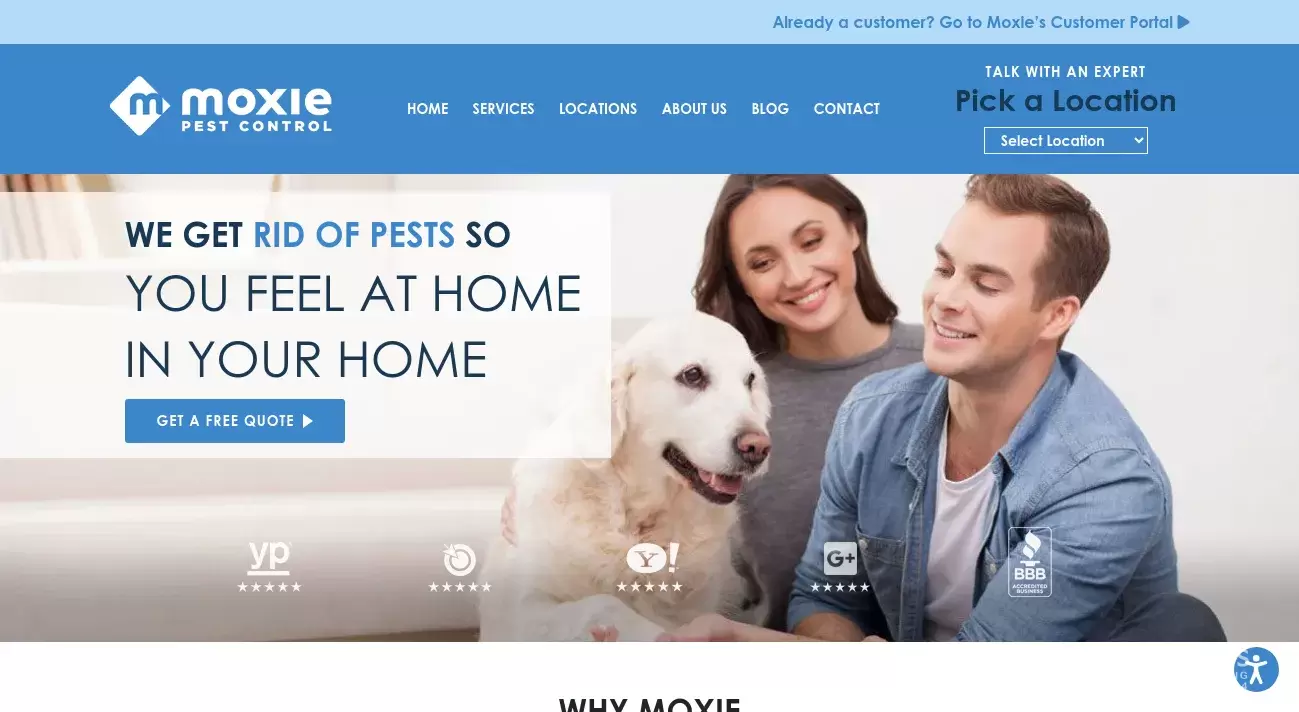This is a screenshot of a website titled "Moxie Pest Control." The title, "Moxie Pest Control," is prominently displayed in white text against a medium blue bar that spans the top of the page. Situated on this blue bar are several menu options: "Home," "Services," "Locations," "About Us," and "Blog." Additionally, there is an option on the right side of the bar that allows users to select a specific location they want to research.

Occupying the main part of the webpage is a photograph featuring a young man and a young woman, both smiling and holding a white dog. Below the photograph, a tagline reads, "We get rid of pests so you feel at home in your home." Positioned at the very top right corner of the page is a button labeled "Customer Login," providing users with quick access to their accounts.